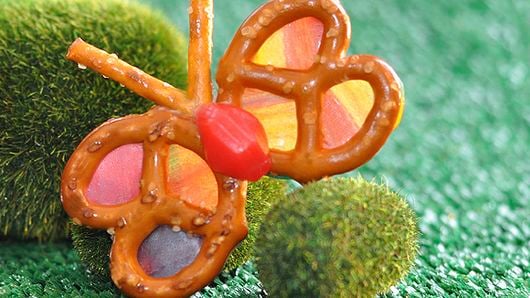The photograph showcases an intricately crafted butterfly sculpture made of pretzels. The butterfly's wings are formed by two full-sized pretzels, while two pretzel sticks represent its antenna. At the center is a vibrant orange candy piece serving as the butterfly's body. Nestled within the holes of the pretzel wings are vibrant candy-colored materials in hues of pink, yellow, purple, and blue, enhancing the semblance of wings. Surrounding the butterfly are soft green moss balls of varying sizes, positioned on a felt-like surface that mimics a grassy, golf course texture. The butterfly is propped at a slight diagonal angle against the moss balls, giving the impression of a whimsical, candy-laden creature in a playful, natural setting.